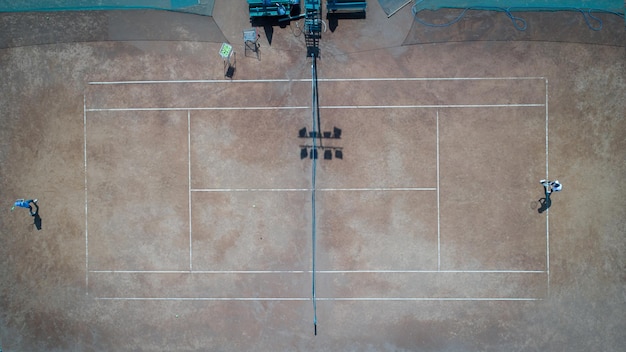This aerial photograph showcases a clay-colored tennis court outlined in white. At the center, a net divides the playing field, though it's somewhat indistinct from this vantage point. On the right side of the court stands a person wearing a white-brimmed hat, while on the left side, another individual is distinguished by a blue head covering, possibly engaged in a match. Behind them, at the back end of the court, are two tall chairs positioned to the left of the net—one green and one blue, presumably for spectators or officials. Just behind these chairs is a black, blue, and green box, likely equipment or storage. Close to the net on either side are two more chairs and an additional black box with green and blue elements. Overhead, several light fixtures can be seen, indicating the court is equipped for nighttime play. The overall view is somewhat distant, capturing both the subtle details and the broader layout of the tennis court.